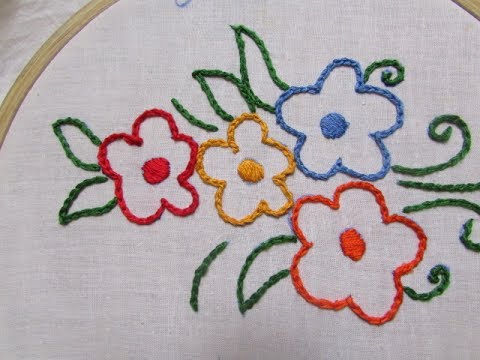This photograph showcases a delicate embroidery on a white cloth, highlighting an assortment of four colorful flowers. Each flower features a simple outline with five petals and a thicker central fabric. The flowers are stitched in red, yellow, blue, and orange threads. Surrounding them are basic green outlines of leaves and stems. The white cloth, which serves as the background, is attached to a light brown wooden surface, portions of which are visible at the top left and top right of the image. The embroidery appears uncomplicated, resembling a needlepoint design that one might hang on a wall as a decorative piece.